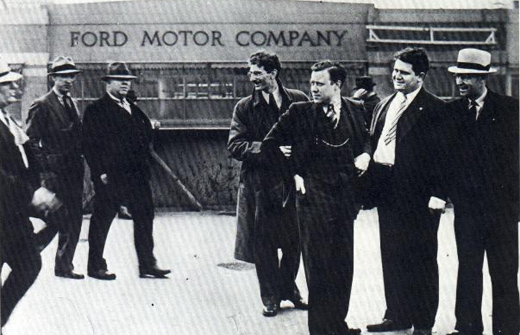In this early 20th-century photograph, likely from the 1920s, a group of seven men gather in front of a gray wall inscribed with "Ford Motor Company" in dark gray letters. The image is rendered in classic black and white, emphasizing the contrast and attire of the period. Four men are already assembled, dressed in dark suits and some with overcoats, exuding an air of formality and camaraderie. They are captured mid-conversation, smiling warmly. Joining them are three more men, all donning hats that vary in style but share a sense of the era's fashion. The man on the far right stands out with his distinct white hat featuring a gray band. This scene depicts a relaxed, friendly meeting among well-dressed gentlemen, highlighting the professional yet convivial atmosphere of the Ford Motor Company during that time.